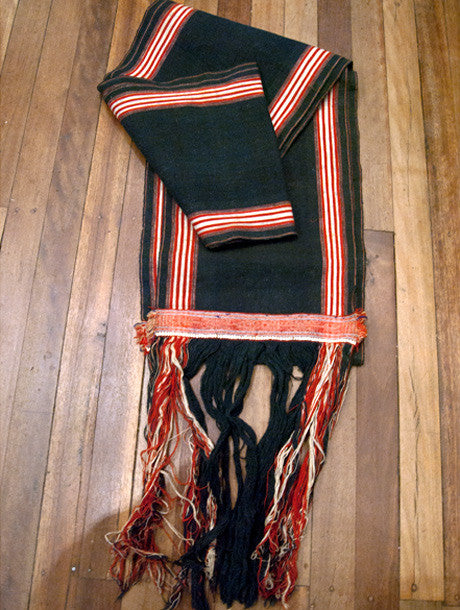The image is a vertical photograph taken indoors, capturing a folded black scarf on a hardwood floor composed of light and dark brown planks. The scarf, which is folded over itself several times at an angle, features vertical red and white stripes along its side borders and a similar border at its bottom edge. The bottom of the scarf also displays tassels in a pattern of red and white on the left and right sides, with solid black tassels in the middle. The perspective is from above, looking directly down at the scarf, which adds a slight shadow at the bottom of the image from the photographer.